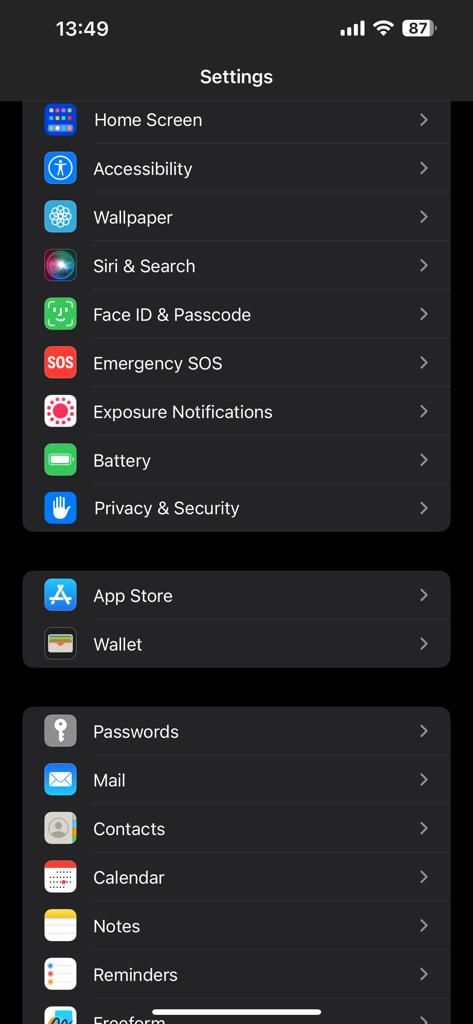The image appears to be a screenshot of a smartphone's Settings menu, captured in portrait orientation. The background is black, providing a clear contrast to the white text and icons. At the very top of the screen, on the left side, the time is displayed as 13:49. On the right side, the battery icon indicates 87% battery life remaining.

Centered at the top, the word "Settings" is prominently displayed, guiding the user through various configuration options. The settings are organized vertically into separate sections, each with distinct options and icons for easy navigation.

The first section lists the following options:
1. **Home Screen** - Icon depicting a stylized representation of the home screen.
2. **Accessibility** - Icon symbolizing accessibility features.
3. **Wallpaper** - Icon displaying a picture frame or image.
4. **Siri & Search** - Icon featuring a microphone.
5. **Face ID & Passcode** - Icon illustrating a facial profile within a frame.
6. **Emergency SOS** - Icon showing a cross or emergency symbol.
7. **Exposure Notifications** - Icon related to health notifications.
8. **Battery** - Icon representing a battery.
9. **Privacy & Security** - Icon often depicted as a lock or shield.

The second section includes:
10. **App Store** - Icon symbolizing a shopping bag or storefront.
11. **Wallet** - Icon often resembling a wallet or card holder.

The final section provides options for:
12. **Passwords** - Icon usually indicating a key or lock.
13. **Mail** - Icon depicting an envelope.
14. **Contacts** - Icon showing a silhouette of a person.
15. **Calendar** - Icon resembling a calendar page.
16. **Notes** - Icon indicating a notepad or document.
17. **Reminders** - Icon likely depicting a checklist or bulletin.

Each option is flanked on the left by a small square icon that visually represents the function, aiding quick identification. On the far right of each option, a small right-pointing triangle suggests that tapping the option will open further settings or additional choices. This user-friendly design assists in easy navigation through various customization and functional features of the device.